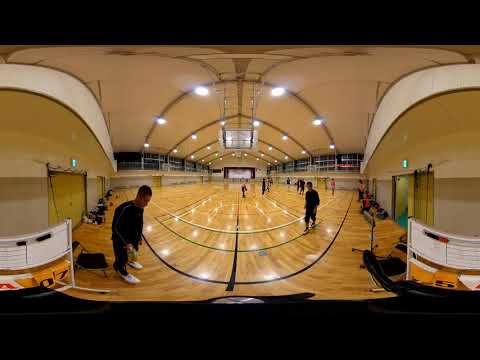This panoramic image, captured with a fisheye lens, showcases a high school basketball court bustling with activity. The court, featuring a pale pine-colored wooden floor, appears wide and clean under the bright, white ceiling lights which create a distinct glare on the floor’s surface. The gymnasium's arched layout, distorted by the fisheye lens, gives the impression of curving lines and circular patterns both in the ceiling and on the court itself. 

A rectangular black border at the top and bottom frames the picture, emphasizing the gym’s elongated perspective. The ceiling, adorned with rows of circular lights, adds to the effect. Down on the court, approximately a dozen young people are seen, some dressed in black outfits, suggesting they might be practicing or preparing for a game in what looks like an open gym setup. The absence of stands hints that no official game is taking place.

On the left and right edges of the photo, white dividers on wheels and emergency exit doors are visible. Toward the back of the gym, a stage and seating area can be faintly discerned, along with people seated against the right wall. Windows lining the top back wall of the gymnasium suggest it is nighttime. Overall, the image captures a vibrant scene of youthful energy within the distinctly lit and structured gym environment.